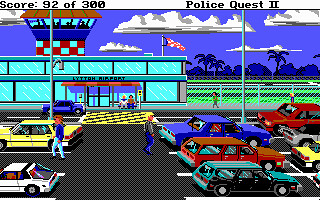The image is a screenshot from an old-style, pixelated video game, likely 8-bit or even earlier, titled "Police Quest 2," as indicated by the text in the top right corner. In the top left corner, a white bar displays the score as 92 out of 300. The scene is set in a brightly colored airport parking lot against a backdrop of palm trees and a mountain range with grassy areas in the foreground. The airport building, distinguished by its neon blue color and red overhang, has a control tower rising from it with a red-and-white checkered pattern and a bulbous top featuring a blue structure with an orange roof.

In the parking lot, there are various damaged cars with smashed windows. On the left, a small white car and a yellow car occupy spaces with an open spot between them. Across from them sits a purple muscle car, also showing signs of broken windows. Further to the right, two station wagons, one red and one blue, are similarly damaged. Near the center, two figures stand facing away from each other: one has blonde hair, a gray shirt, and blue pants, while the other has brown hair, a blue shirt, and light tan pants. Additional cars can be seen in the extended section of the parking lot to the right. The overall atmosphere of the scene is vividly retro and chaotic, capturing the essence of vintage gaming aesthetics.